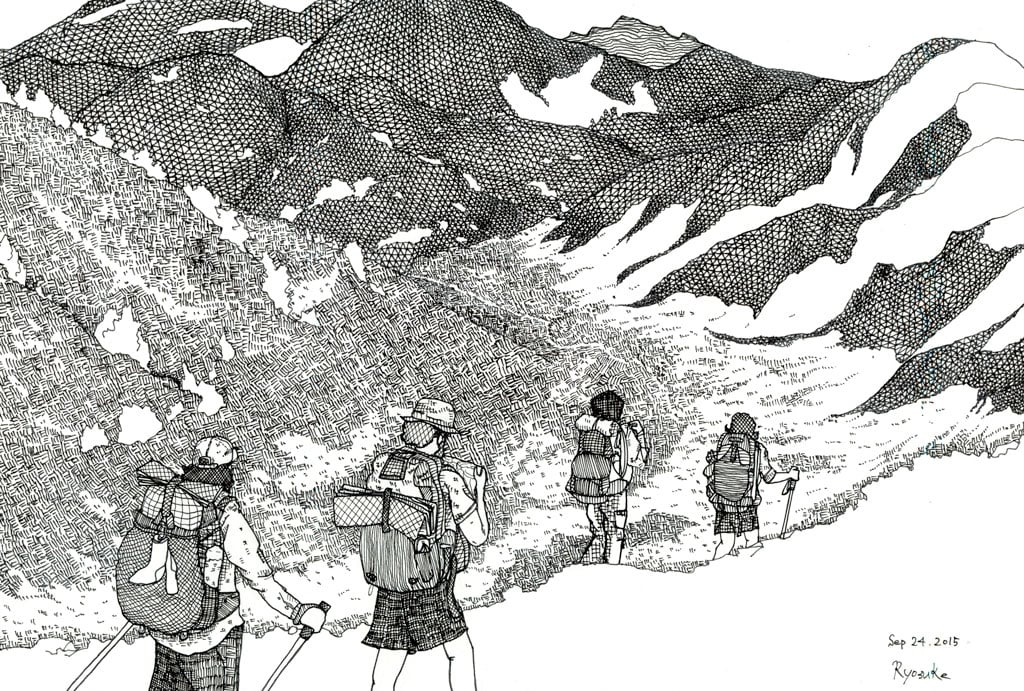The black and white illustration, dated September 24th, 2015, and signed by Ryosuke, vividly captures an outdoor scene of four hikers trekking along a mountainous path. The mountainous backdrop stretches from the top of the image to the center, showcasing dark grey, snow-capped peaks etched in a crisscross pattern. The snow is stark white, covering both the lofty peaks and parts of the valley below. 

In the foreground, the hikers, clad in shorts and equipped with backpacks, are depicted from the back. Two of them also sport hats. The group appears to be led by a woman, followed by another woman, who is holding a walking stick. The third hiker, who might be a man, is engrossed in reading a map and is not holding a stick. The last hiker, probably another man, is equipped with two walking sticks and has a pair of socks dangling from his backpack. The hikers' journey, through a snowy, rugged terrain, conveys a sense of adventure and determination as they ascend the mountainous trail.